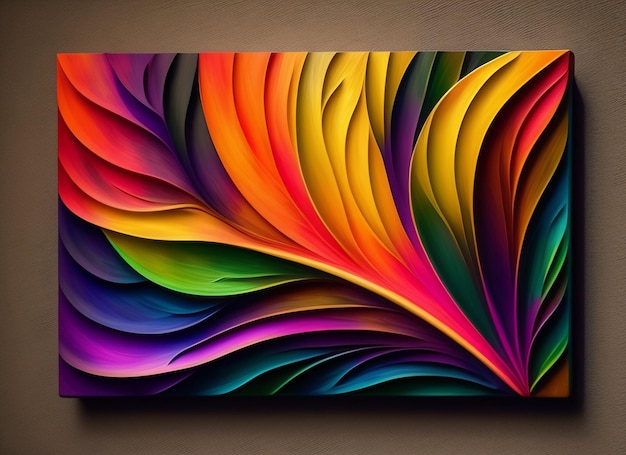This image showcases a rectangular canvas painting, set against a textured brown-gray wall that seems tangible enough to touch. The artwork, vibrant and highly detailed, portrays an impressionistic botanical design. It features a central vein with smaller veins extending outward, resembling either leaves or feathers intricately layered over each other. The painting dazzles with a rich spectrum of colors—yellow, purple, orange, green, blue, pink, turquoise, and red—creating a seamless blend and fade across the surface. The thick, textured paint or possibly digital rendering gives the painting a three-dimensional effect. The positioning of the artwork casts notable shadows to the right and bottom, indicating it is hung inside, and adds depth to the overall composition.